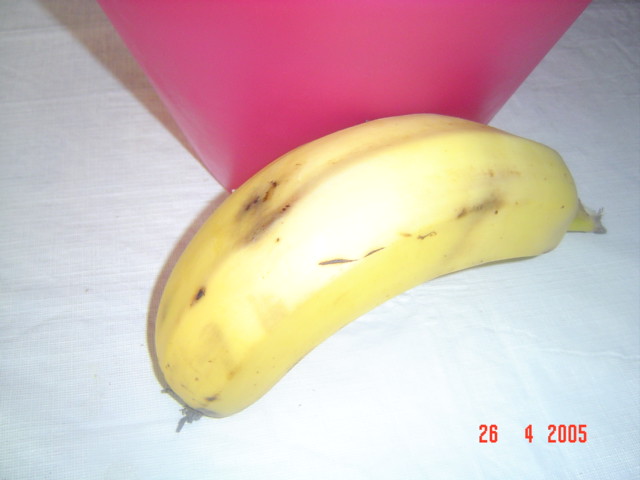This image captures a plump and unusually short banana positioned on a white cloth. The cloth extends across the frame from the top to the bottom, running horizontally from left to right. Subtle shadows grace the top left and right corners, while a bright light source from below illuminates the banana, casting it in highlight.

The cloth, with its wrinkles traversing from left to right, forms a textured backdrop. Approximately an inch from the left side, a dark pink plastic tub enters the frame. This tub descends diagonally to the right, disappears behind the banana, and then reappears before exiting the frame about an inch from the right side. The tub's shadow is visible on its left side.

The banana sits prominently in the midst of this setting. Its top, meant for peeling, is oriented toward the right, just an inch from the edge. It curves in front of the pink tub and then gently arcs to the bottom left, creating a slightly angled lower segment. This banana, notable for its thick and stout shape, shows signs of bruising near the pink tub and along its right side.

In the bottom right-hand corner, the date "26 4 2005" is inscribed in red, adding a timestamp to the scene.